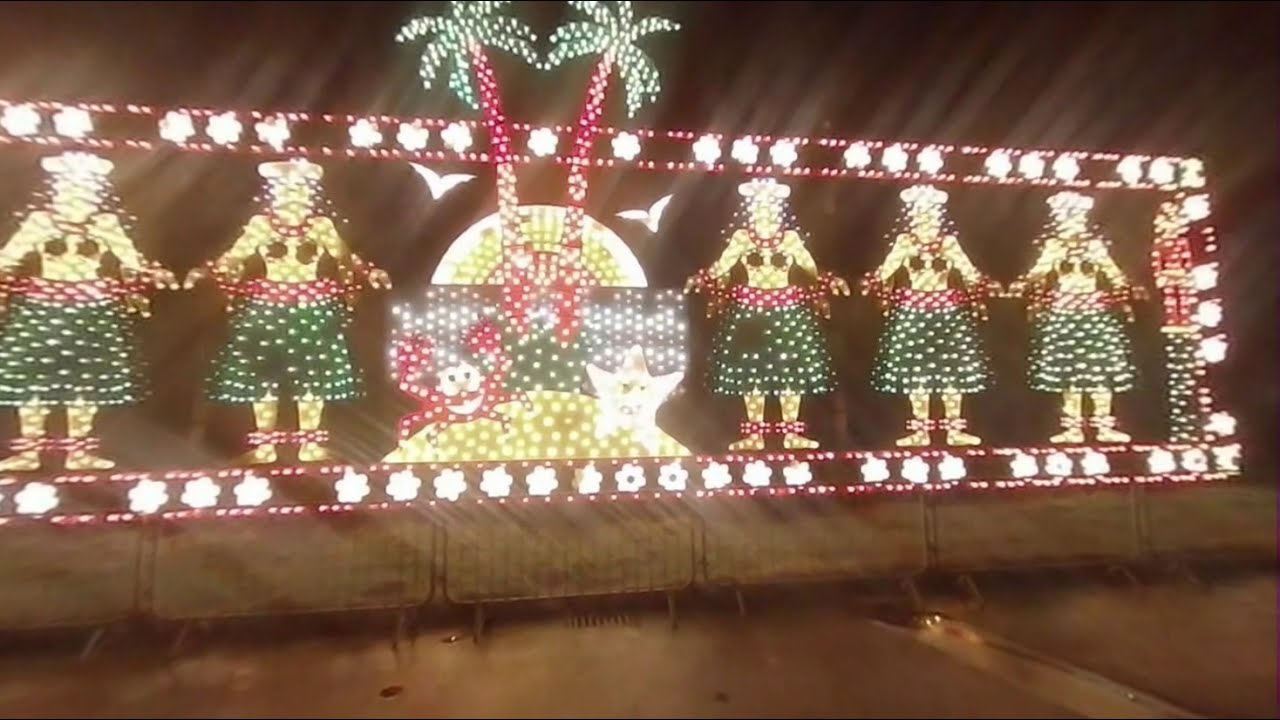This illuminated display features a vibrant Christmas theme set on a tropical island, most likely Hawaii. The billboard is rectangular and bordered by glowing lights, with an intricate outline of what appears to be flowers. The border features multiple glowing stars. Dominating the center are two palm trees made of lights, boasting red trunks and green leaves, flanked by a yellow star at the base, and a red crab on the left. On the right side of these palm trees are three illuminated hula dancers, while two more stand to the left, all dressed in green skirts, red belts, and coconut-style bikini tops. The dancers also feature detailed white-lit head wreaths. The entire scene is set against a red horizontal backdrop, giving the display a festive and tropical ambiance.